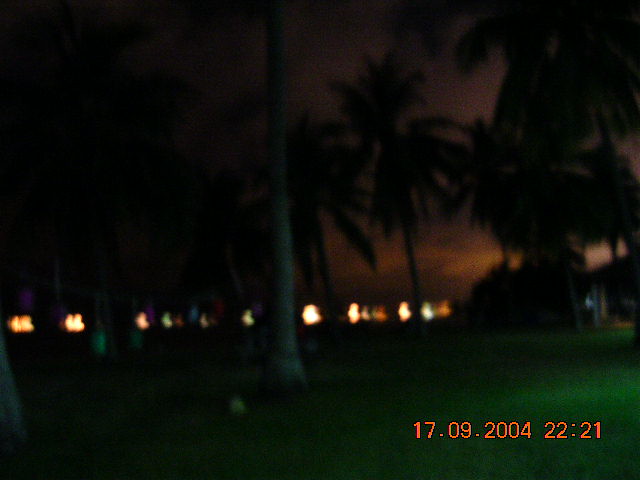A low-resolution, blurry image in a square format captures an outdoor scene featuring several tall palm trees standing on a grassy field. The trees reach towards a sky rendered in shades of black and orange, possibly suggesting a sunset or a photographic filter. The scene is poorly defined due to the fuzzy quality of the picture, making details difficult to discern. At the bottom of the image, an orange timestamp reads "17.09.2004 22:21," indicating the date and time the photograph was taken.